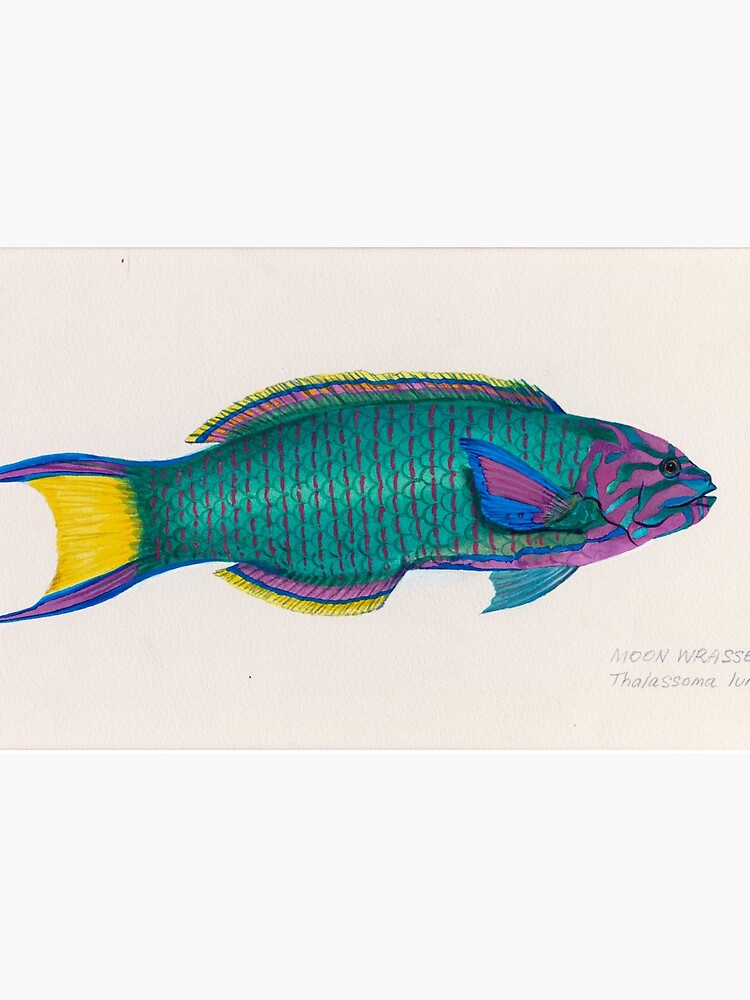The image is a detailed drawing of a fish centered on a slightly pinkish-tan rectangular piece of paper, roughly five to six inches high and four inches wide, framed by light gray borders along the top and bottom thirds. The fish, oriented head to the right and tail to the left, is depicted with precise coloration: its main body is a cyan or teal blue with light blue scales and vertical dark purple or pink lines running down it. The face primarily features a mix of light blue and purple lines. The fish's tail fin showcases a pattern with dark purple edges transitioning to blue, and connecting yellow tips. The long fins on the top and bottom of the fish exhibit a gradient from purple to blue to yellow. The side flippers are outlined in blue with a purple interior. Inscribed in pencil at the bottom right of the image are the partially obscured words "Noon," "Wrasse," and "Thalassoma," with additional letters cut out of view.